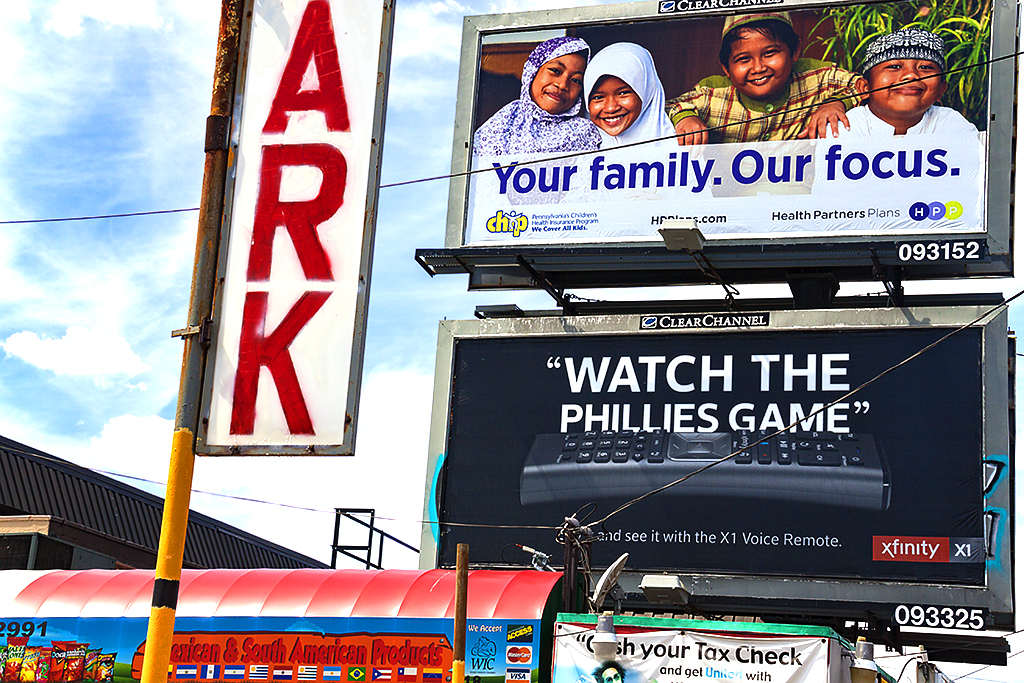In the image, there are multiple signs prominently displayed:

1. The top billboard features an advertisement for Health Partner Plans. It showcases a diverse, dark-skinned Asian family composed of four individuals. The slogan "Your Family, Our Focus" is written in blue text, emphasizing the company's commitment to family-centric healthcare.
   
2. Below this, another billboard invites viewers to "Watch the Phillies Game." This ad, which is primarily in white text on a black background, includes an illustration of a keyboard. It promotes Xfinity services with the code "XI 093325" mentioned beneath the ad.

3. At the bottom, a smaller sign reads, "Cash Your Tax Check," indicating a place where financial transactions such as cashing tax refunds can be conducted. 

All the signs are arranged vertically, each with distinct purposes and target audiences.